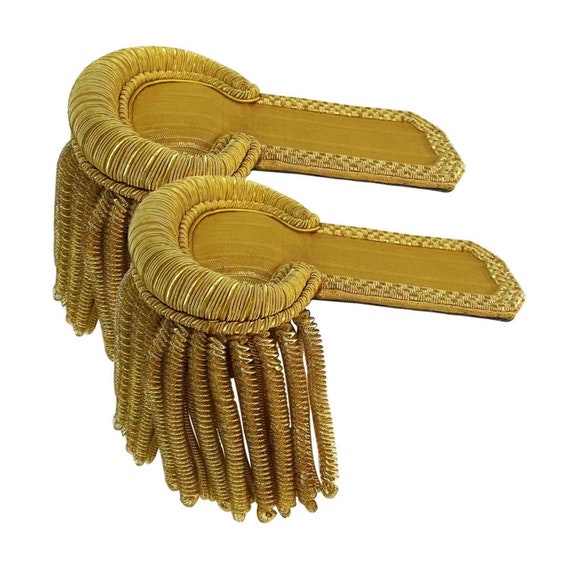The image depicts a bright, clear close-up photograph with a solid white background, showcasing two golden fabric objects aligned next to each other. These objects have a distinctive rectangular shape on the right side, transitioning to a rounded shape on the left edge. Encircling each rectangular end is a decorative, stitched border that appears more elaborate and textured, resembling a thin croissant or rope pattern. Inside these borders, the fabric is smooth and solid in color, highlighted in golden tones. At the rounded end of each object, a bunch of tassels made from coiled and twirled fabric dangle prominently. These tassels, resembling cylindrical, dark brown ropes, cascade down from the edges, giving the objects an ornate and detailed appearance. The image is devoid of any text, borders, or additional objects, focusing solely on the intricate design of the golden fabric pieces.